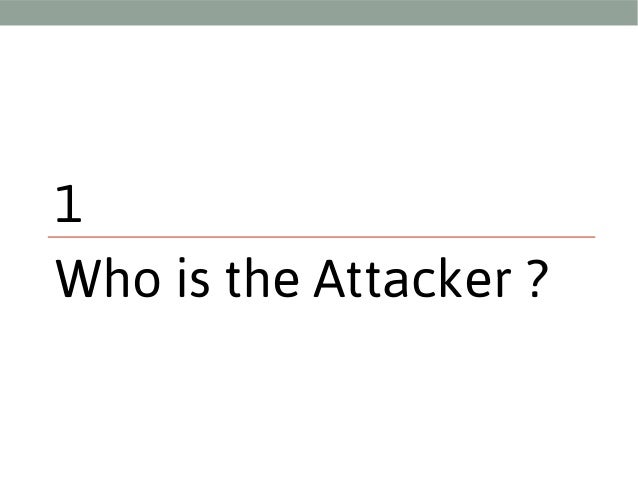The image is a simple presentation slide with a white background. It features a gray horizontal border at the top. Centrally aligned, the text begins with the numerical "1" in black font. Beneath the number is a thin red horizontal line, followed by the question "Who is the attacker?" in black font, with "W" and "A" capitalized and ending with a question mark. All elements are centered and there are no other visuals present on the slide. The overall design is minimalistic, focusing solely on the text and lines.